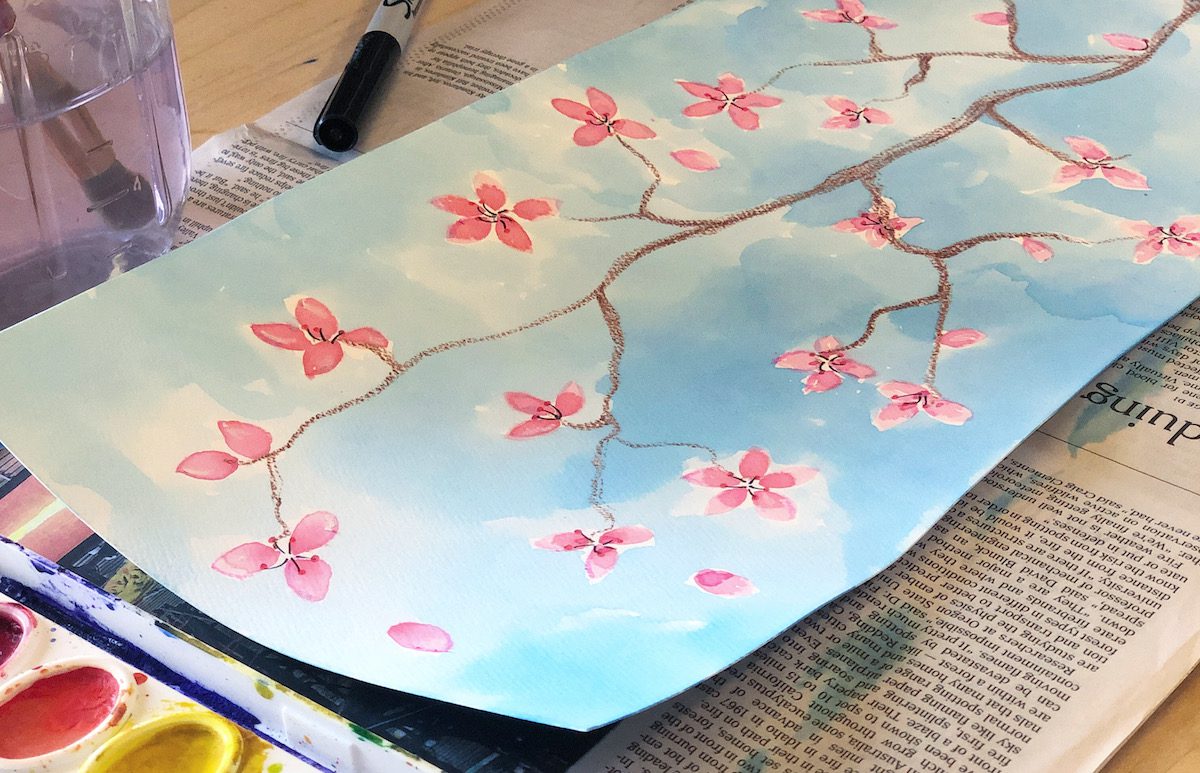The image shows an intricate watercolor painting that is positioned on a wooden table covered with newspaper. The painting, created on a long rectangular sheet of white paper, depicts a beautiful branch of cherry blossoms. The delicate flowers, varying in shades of pink and red, bloom from a thin brown vine. The background features a blend of light and dark blues, resembling a serene sky or water. In the scene, various art supplies are visible: a Sharpie marker on the left side, a palette in the bottom left corner with red, yellow, and purple paint, and a jar of water holding a brush. The overall setup provides a glimpse into an indoor art session, capturing the essence of creativity and meticulous detail in the artwork.